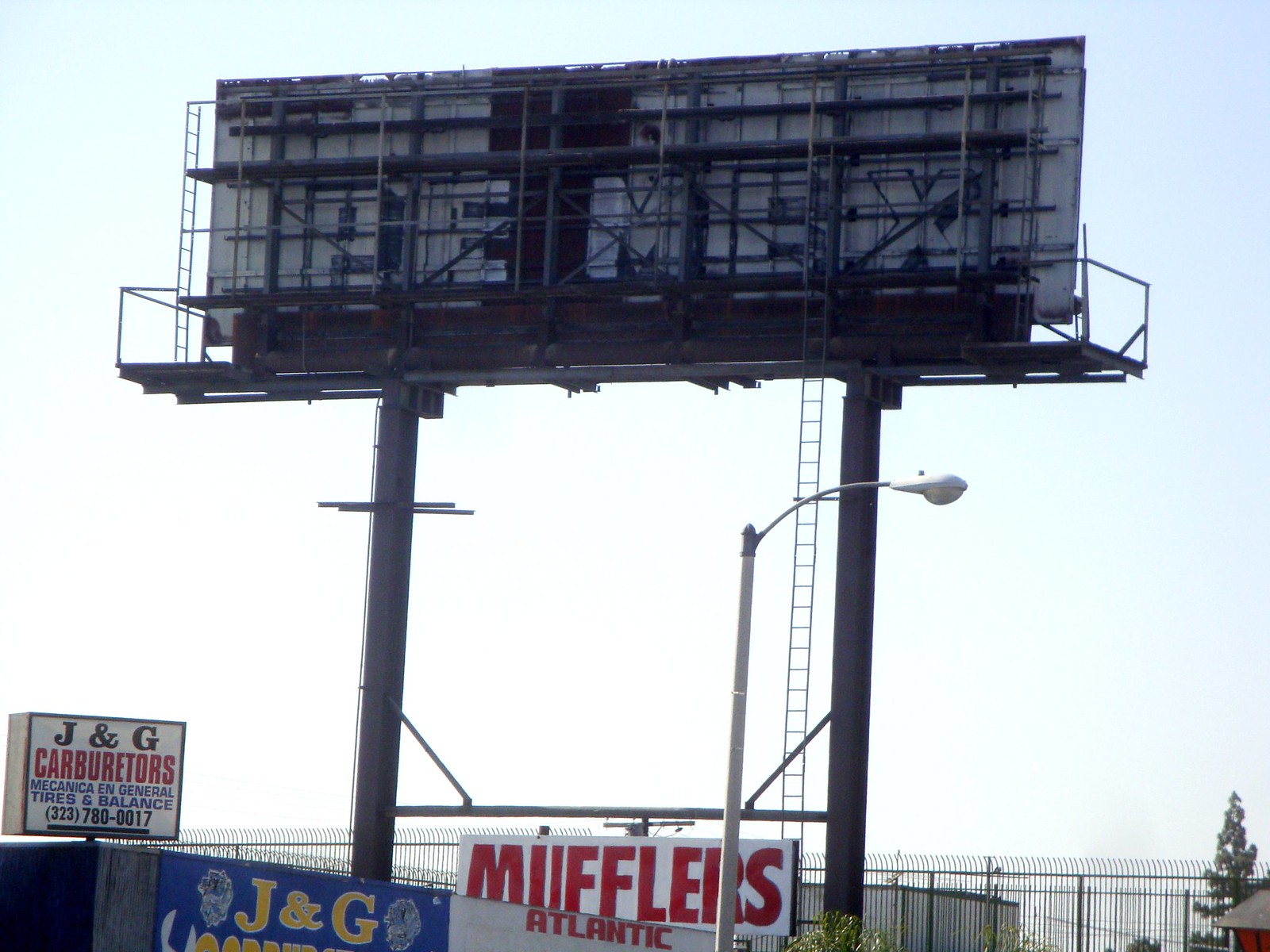The photograph captures an outdoor scene featuring a vibrant cyan blue sky that fades to white at the horizon. Dominating the image is the backside of a large white billboard, supported by silver beams and dark gray poles, and encircled by a dark gray safety railing. Below the billboard, a tall black metal security fence with thin vertical bars and curved tops sits at the forefront, likely designed to deter climbing. Attached to this fence are several business signs: on the left, a rectangular sign in white reads "J & G Carburetors," accompanied by a phone number, "323-780-0017," and additional services in both Spanish and English. Nearby, another sign in yellow and blue also bears the name "J & G," while a third sign below the large billboard features "Mufflers" in bold red letters on a white background. There is also a smaller sign with "Atlantic" in bold capital letters. The backdrop includes evergreen trees and warehouse-like metal buildings, with a tall street lamp and long ladder extending from the billboard down to the ground, enhancing the industrial ambiance of the scene.